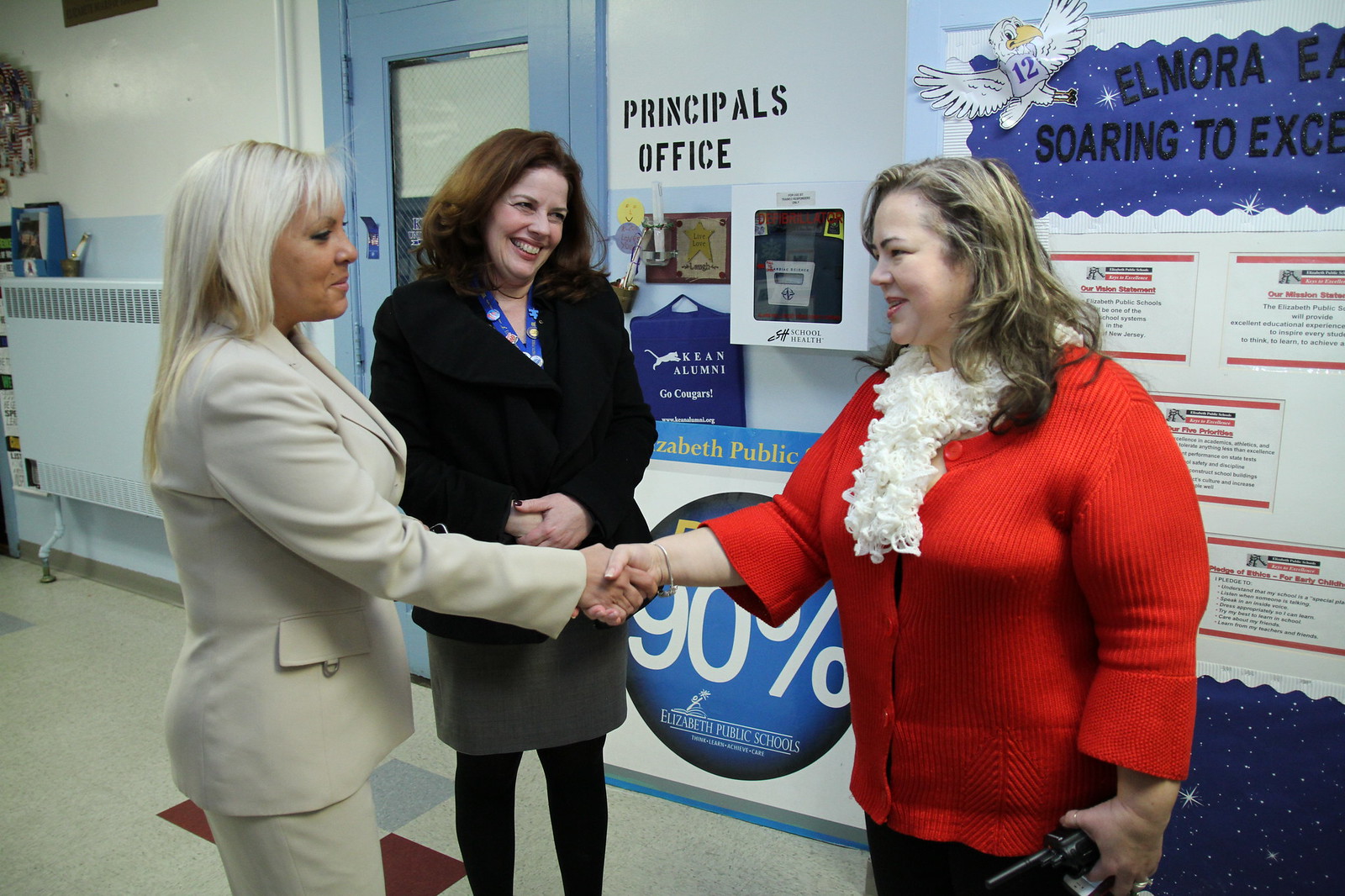In this image, three women are greeting each other in a school setting, identifiable by the sign "principal's office" and a wall-mounted defibrillator nearby. The woman on the left, dressed in a beige business suit with bleached white hair, is shaking hands with a heavyset woman on the right who wears a red sweater, a frilly white scarf, and holds a walkie-talkie. Positioned between them is another woman dressed in a black blazer and skirt, smiling warmly at the woman in red. The backdrop features light blue striped walls and a door with a light blue frame and clear glass center, suggesting they are right outside the principal's office. The word "Elmora" appearing in the background likely indicates the name of the school.